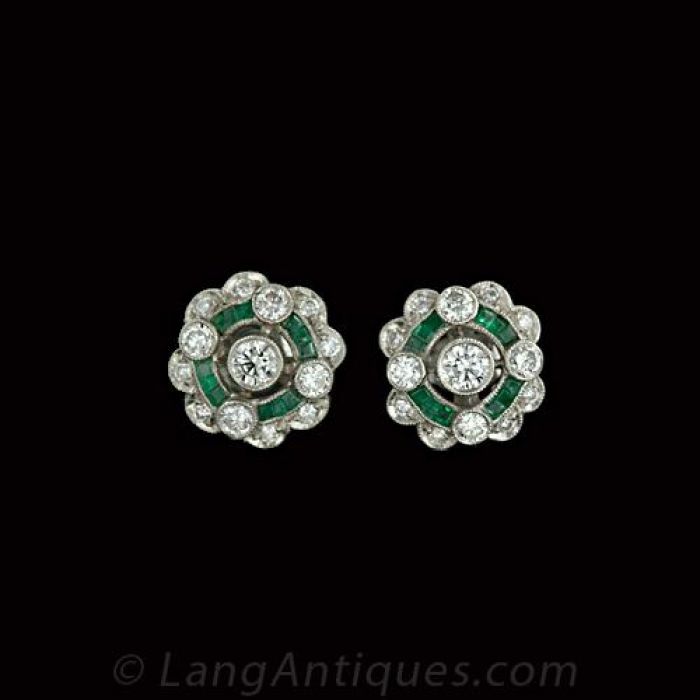This image, courtesy of LangAntiques.com, showcases an exquisite pair of antique diamond and emerald earrings set against a stark black background. Each earring prominently features a large round diamond at its center, encircled by a row of princess cut or baguette emeralds. Within this vivid green layer, four additional diamonds are interspersed, each positioned at the cardinal points. Surrounding the emeralds is yet another outer ring of eight round diamonds, creating a stunning, clustered effect. The contrast between the sparkling diamonds and the lush green emeralds is strikingly highlighted by the dark background, ensuring the intricate details and brilliance of these heirloom pieces are impeccably showcased.